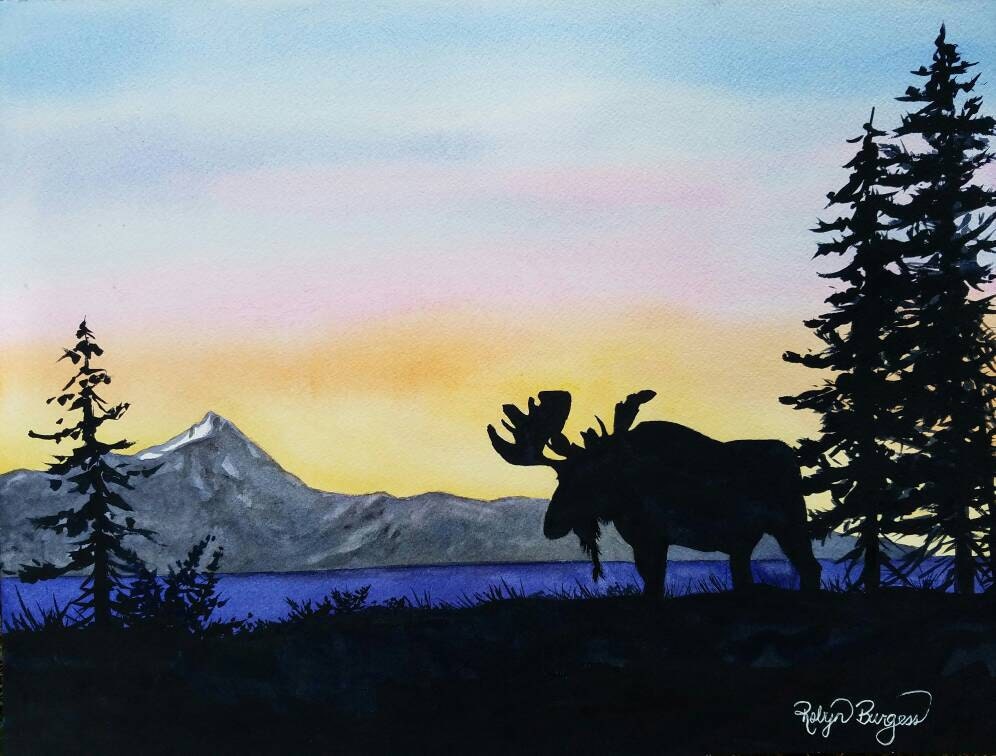This painting, signed by the artist Robin Burgess in white cursive in the bottom right-hand corner, depicts a serene nature scene centered around a majestic moose with large antlers. The moose stands off-center on a grassy patch, facing left, surrounded by three fir trees—two behind it and one in front. The background features a gray stone mountain and a tranquil blue lake, both adding depth to the landscape. The sky above is a beautiful gradient of watercolors, transitioning from yellow near the mountains to orange, pink, and then blue at the top, with a slight hazy, cloudy texture. The overall composition elegantly captures the peacefulness and majesty of the natural world.